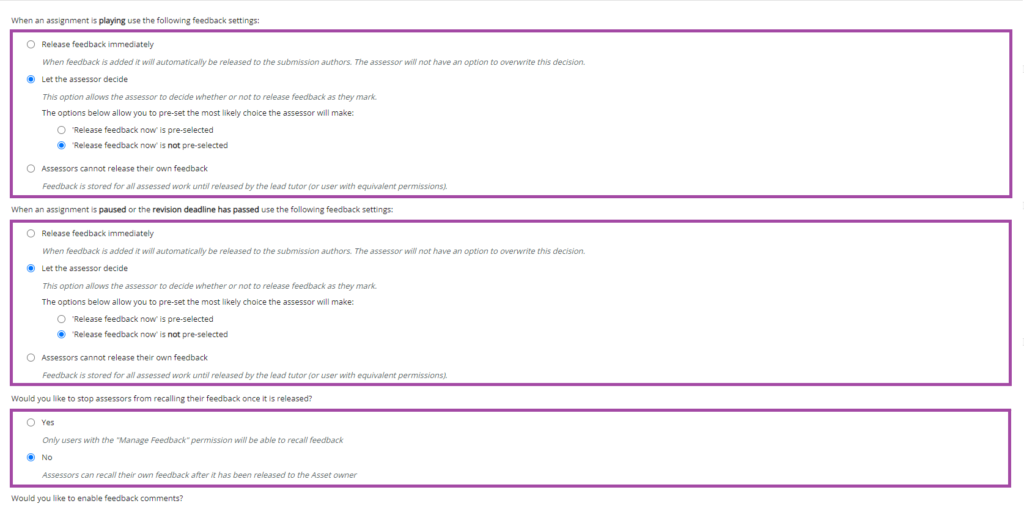A cropped screenshot from a web page depicts a section of information, primarily a settings menu for an online assessment tool. The image features a white background with dark grey text, organized into four distinct questions, each followed by radio button options enclosed with a purple outline. 

1. The first question reads, "When an assignment is playing, use the following feedback settings," accompanied by a list of setting options selectable via radio buttons.
2. The second question asks, "When an assignment is paused or the revision deadline has passed, use the following feedback settings." This section also includes radio button selections.
3. The third question inquires, "Would you like to stop assessors from recalling their feedback once it is released?" Here, users can choose between two radio buttons labeled "Yes" and "No."
4. The final question at the bottom asks, "Would you like to enable feedback comments?" with a similar yes or no radio button option available.

The layout is clear, focusing solely on the settings configuration for an online assessment, with no web browser, address bar, or website header details visible in the screenshot.